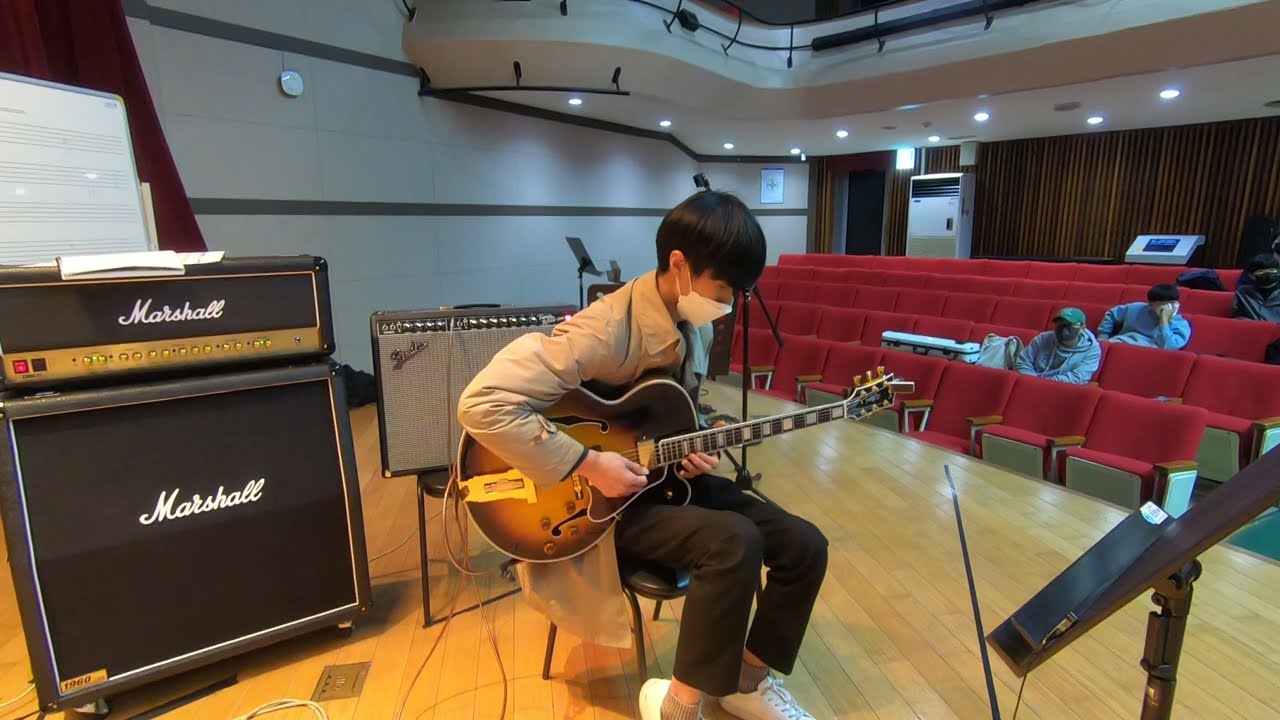This highly detailed photorealistic image portrays a young boy, approximately 12 years old, seated in a central position on a light yellow wooden stage within a small auditorium. The boy, who has short black hair, is looking down and strumming a brown electric guitar held under his right arm. He is attired in a gray hooded shirt, black pants, and white sneakers, and he wears a white facial mask. The framing captures his knees pointed to the right side of the image. Behind him on the left stands a prominent black Marshall amplifier stack, comprised of two units, and to its right rests a gray speaker.

To the bottom right of the image is a black music sheet holder. The auditorium features about six ascending rows of red theater-style seats on the right-hand side, occupied by a few individuals, some of whom are wearing gray sweatshirts and using cell phones. The room's walls and ceiling are white, with stage lighting overhead. The top right of the image reveals a large second-story balcony overlooking the stage, bordered below by a dark curtain.